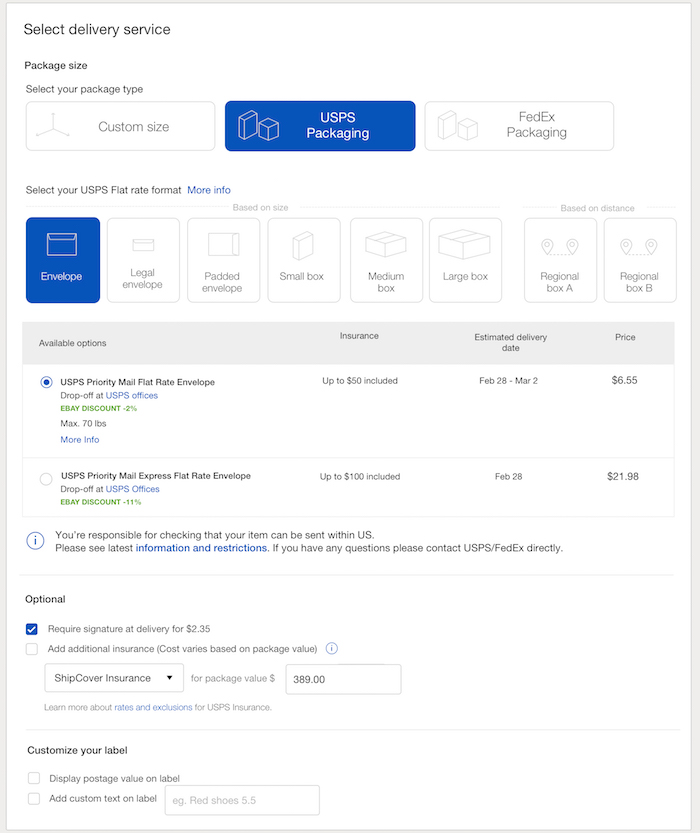This image is a screenshot of an online USPS delivery service selection page. The background is predominantly white with gray and black text. In the upper left corner, the heading "Select Delivery Service" is displayed. Below this, there are various options available, one of which is "USPS Packaging," highlighted in blue, indicating it has been selected. 

On the left side of the page, there are images of different types of boxes. Directly below this section is another option titled "Select Your USPS Flat Rate Format," where "Envelope" has been chosen, turning that button blue.

Further down the page, the option "USPS Priority Mail Flat Rate Envelope" has also been selected, with the note "Drop off at USPS offices" next to it. A green text indicates an "eBay discount minus 2%" off the standard rate, with a maximum weight allowance of 70 pounds. 

Under the "Optional" section, there is a blue checkmark next to "Require Signature at Delivery" for a fee of $2.35. The overall context of the image suggests it is a detailed page used for setting preferences and providing selections for shipping an item purchased online.